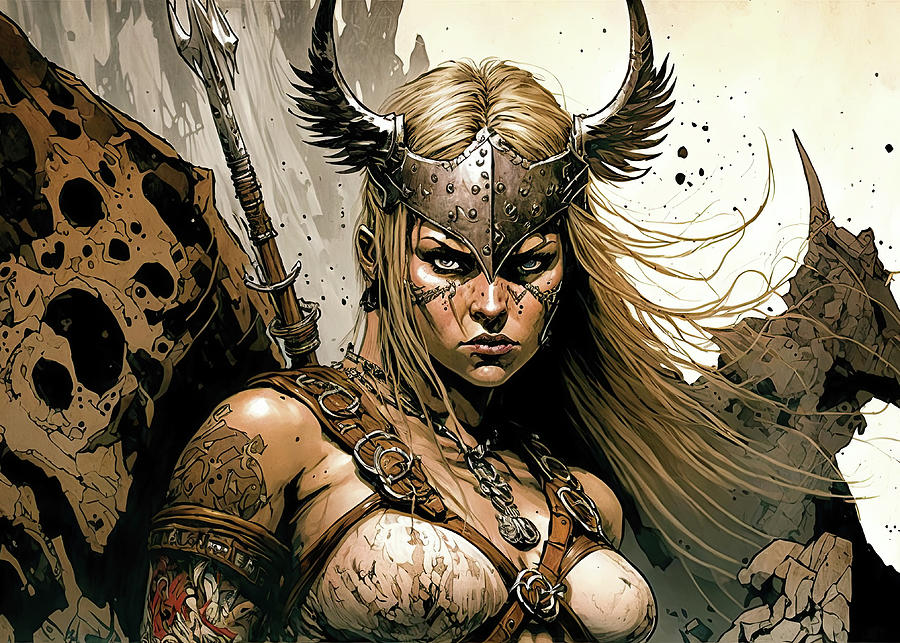The image portrays an animated drawing of a fierce female warrior combining medieval and dystopian elements. The character, drawn from the chest up, wears a brown battle vest adorned with chains and a yellow strap crossing her chest and arms. She has a helmet piece on her forehead, styled with two horn-like feathers, partially revealing her blonde hair. Her piercing gaze is directed forward, exuding determination. A weapon, possibly an axe, spear, or sword, is slung over her shoulder. The setting appears to be rocky terrain, potentially depicting a mountaintop or cave with natural light illuminating the scene. The background transitions from an off-white and beige rocky texture to a reddish sky on the right, enhancing the dramatic atmosphere. The entire image is vividly colored and highly detailed, focusing on this formidable female warrior against a rugged and bright backdrop.